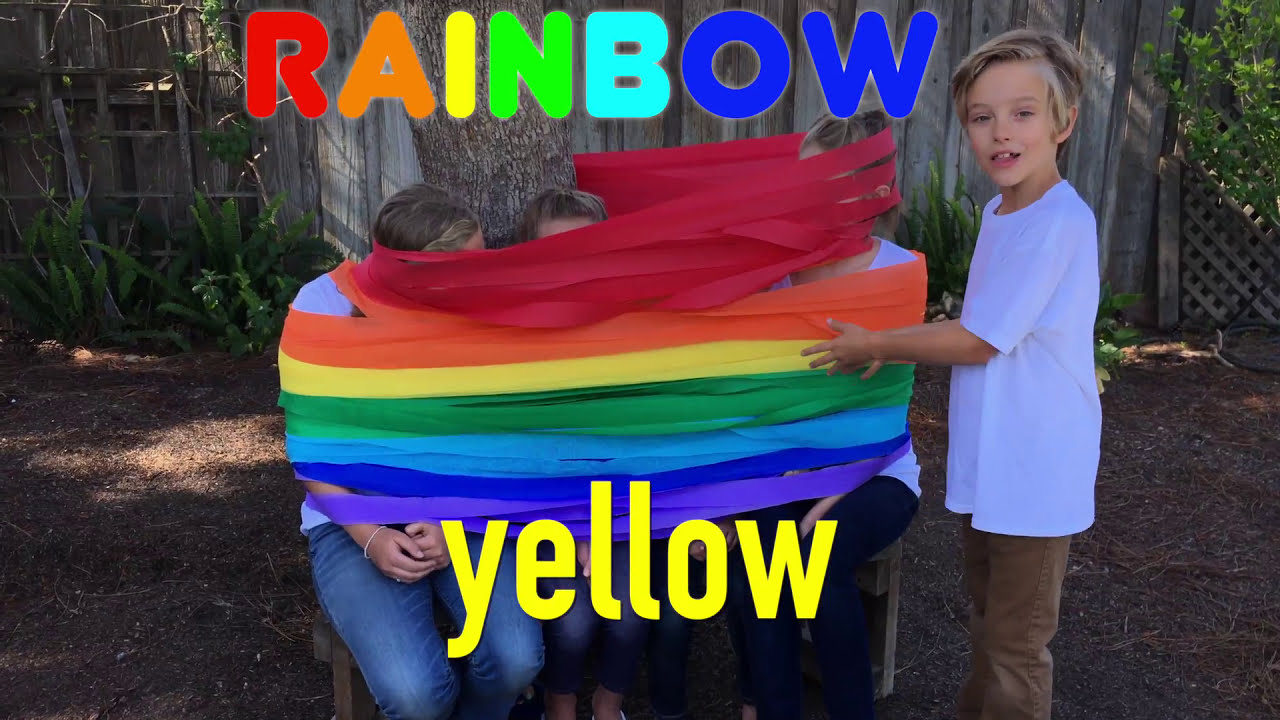The photo depicts a diverse family group engaged in a playful outdoor activity, set against the backdrop of a wooden fence and plants in a backyard. Central to the image are four individuals, likely a mix of young adults and children, seated on a bench next to a tree. They are wrapped in vibrant ribbons in the colors of the rainbow—red, orange, yellow, green, light blue, dark blue, and purple—covering their faces and bodies down to their waists. Above the group, the word "RAINBOW" is prominently displayed, each letter in corresponding rainbow colors. Below the ribbons, the word "yellow" appears in the same hue. To the right stands a small boy with light brown blonde hair, dressed in a white t-shirt and tan pants, who is facing the camera with one arm extended towards the ribbon-wrapped group, fingers splayed. The scene is set on dried brown soil, with no grass visible, and radiates a sense of whimsical fun and family bonding.